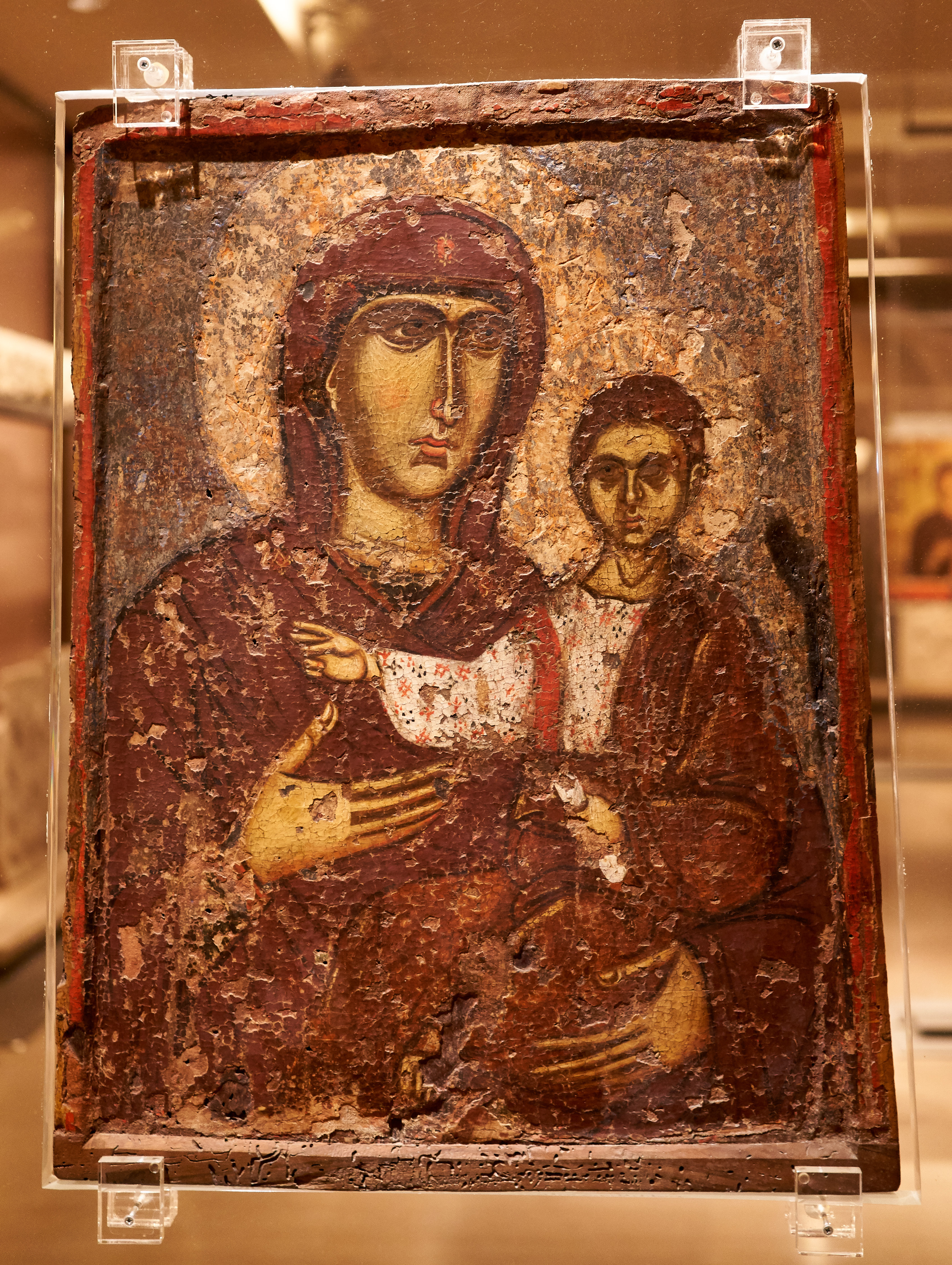The painting, displayed in a museum or gallery setting and protected under an acrylic case, depicts a religious scene with a mother figure, likely Mary, and her child, possibly Jesus. The central figures are rendered with a palette dominated by maroon, brown, and white hues, conveying a sense of antiquity and worn authenticity through visible gouges and imperfections on the surface, which resembles wood or stone.

The mother, positioned on the left, wears a maroon robe with a matching head covering, and is adorned in a traditional dress. Her gaze is tenderly directed toward the child in her lap. Her long, slender fingers encapsulate one hand on her chest and another enveloping the child. The child, swathed in a brownish-red robe over a white upper garment accented with pink and brown markings, holds a rolled-up scroll in one hand. His other hand is at chest level, and he faces forward, creating a poignant connection with the viewer. Both figures are encircled by a halo of light, enhancing their sanctity. The background, with its muted tones, suggests an antiquated, possibly stone-like texture, adding to the painting's historical and spiritual resonance.